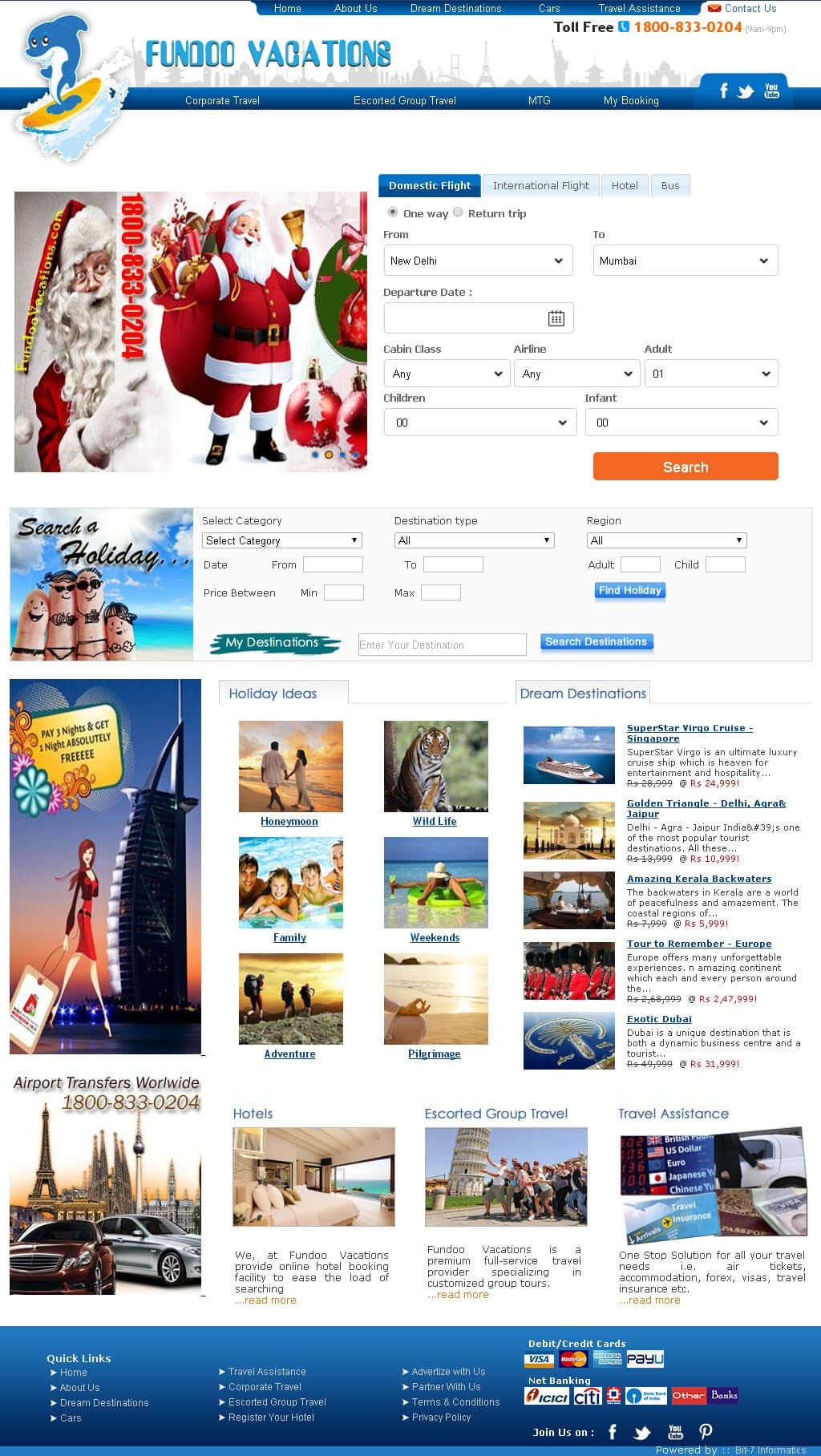This image is a screenshot of a website titled "Fun Odd Vacations," identifiable by its title and logo positioned in the top left-hand corner. The logo features a whimsical cartoon of a shark standing on an orange surfboard. The website itself has a white background and exhibits a variety of eclectic images. In the top left, there's a picture of Santa Claus, while other images scattered across the page include drawn characters on fingers, a woman carrying a shopping bag, two cars parked together, a couple walking on a beach, a tiger, and a small group of people in a swimming pool. In the bottom right-hand corner, icons for different payment methods, including Visa, Mastercard, and American Express, are displayed.